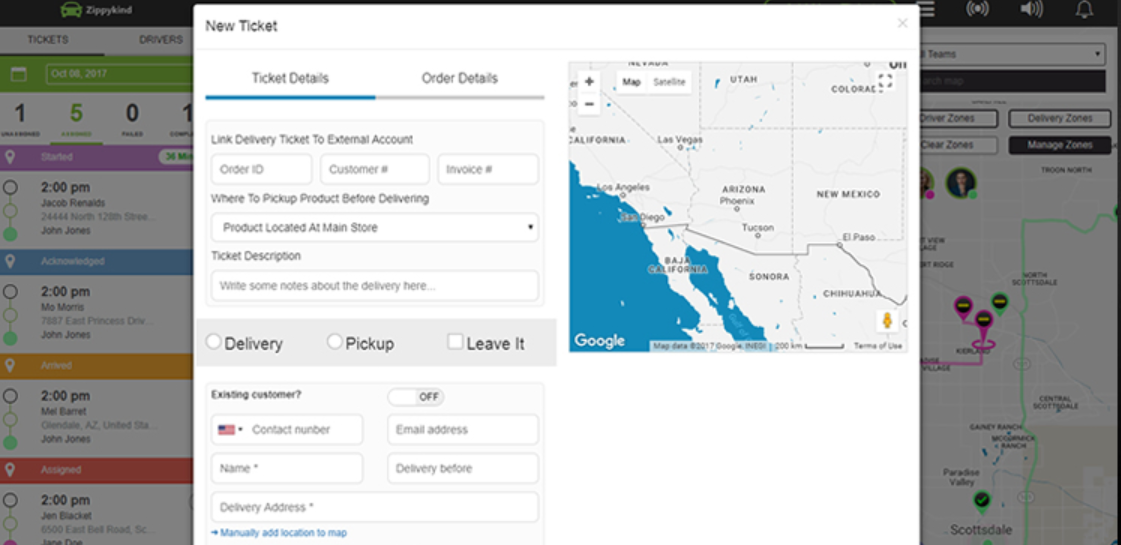The image appears to be a high-resolution screenshot of a website, albeit slightly blurry and not fully in focus, labeled "Zippy Land" in the upper-left corner. The background of the image displays various statuses such as "started," "acknowledged," "arrived," and "assigned," alongside different names and street addresses, with additional names listed below.

In the foreground, a column features sections titled "New Ticket," "Delivery Details," and "Order Details," each containing various pieces of information. To the right, there is a map showing multiple states, including Mexico, New Mexico, Arizona, California, Nevada, Utah, Colorado, and part of Texas.

On the left-hand side, there are details under headings like "Ticket Details," "Delivery Ticket," "External Account," "Order ID," "Customer Number," "Invoice," and instructions on where to pick up the product before delivery, with a drop-down box stating "Product located at main store."

Further sections include "Ticket Description" with a prompt to write notes about the delivery, "Delivery" with options for pick up or leave it, and "Existing Customer?" followed by contact information fields asking for a contact number, email address, name, delivery before, and delivery address.